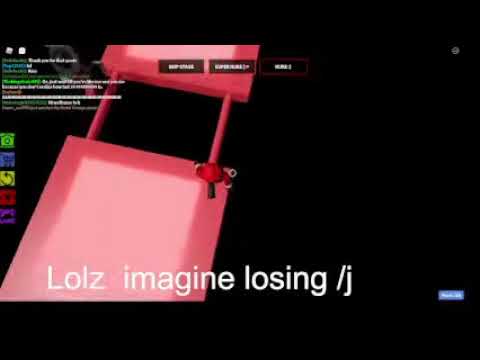The image appears to be a screenshot of a computer screen with an all-black background. Prominently displayed in the bottom left-hand corner is a large pink object, consisting of two interconnected rectangles joined by two small prongs that extend upward. This structure is notably cut off at both the top and bottom edges. In the upper left-hand corner, there is script written in multiple colors—black, blue, green, and brown—spanning approximately seven to eight lines, but it is difficult to discern due to its small size and distance from the viewer. Additionally, the left side of the image features a vertical stack of five colored squares, each possibly representing different icons or functions: green, blue, yellow (notably with a reverse arrow symbol indicating a "go back" action), red, and purple. At the bottom of the image, there is an inscription in white text that reads, "LOLS, Imagine Losing, /J".